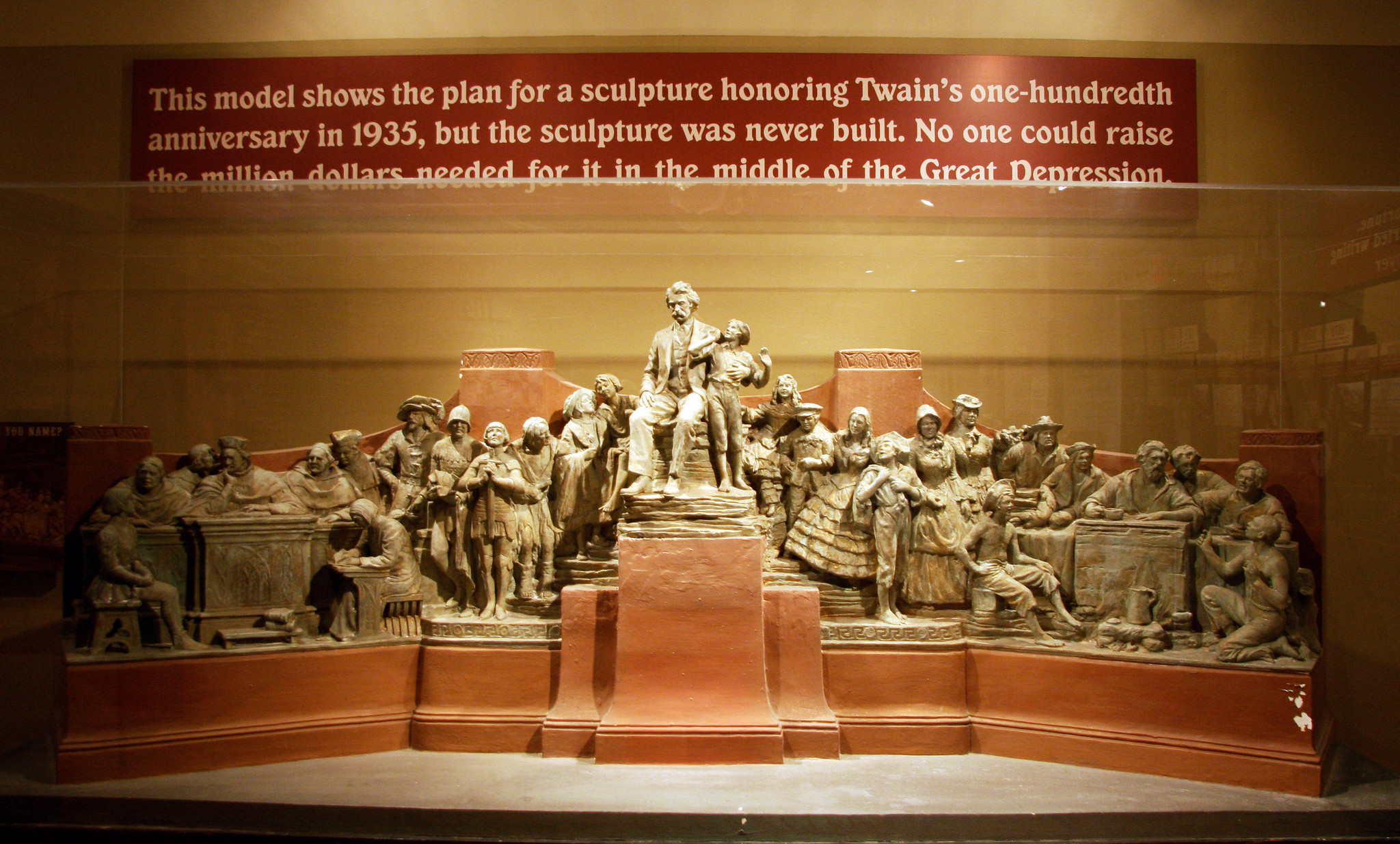This photograph captures an intricate clay scale model of a proposed but never-realized sculpture intended to honor Mark Twain on his 100th anniversary in 1935. The model is encased in glass and features detailed depictions of various figures surrounding Twain, who stands prominently on a raised wooden platform. Twain's arm is around a child, potentially representing Tom Sawyer or Huckleberry Finn, and he is flanked by numerous people in varying poses—some seated or standing at tables and desks, others appearing to be characters such as slaves, rivermen, and possibly his Aunt Molly. The model is primarily grayish-beige and is set against a backdrop with red walls. The accompanying sign explains that the sculpture was never built due to the inability to raise the required one million dollars during the Great Depression. The scene evokes a 1930s setting with figures garbed in period-appropriate attire, including women in long dresses.